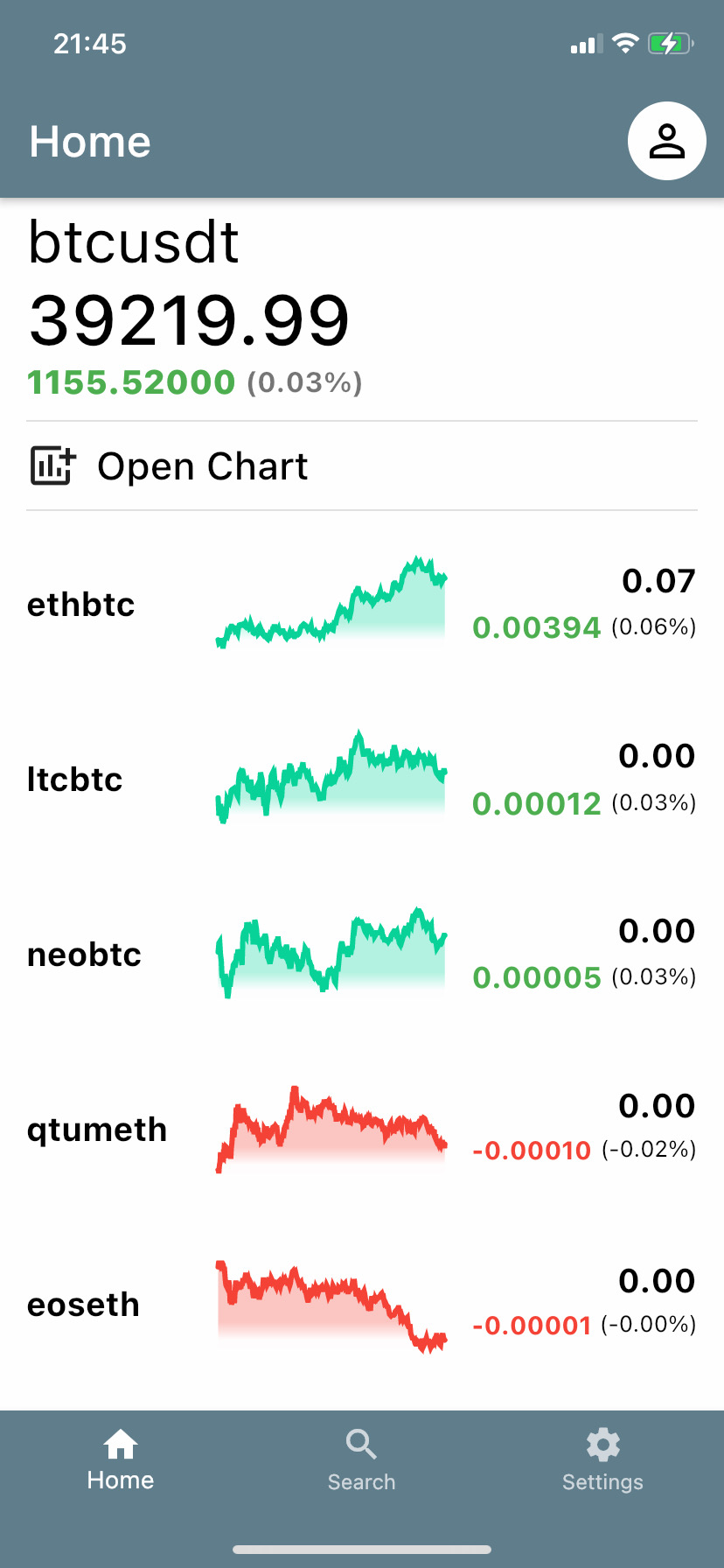The image displays a mobile device screen running on iOS, recognizable by the white horizontal bar at the bottom used for exiting apps. The status bar at the top indicates that it is 21:45 with three out of four cellular reception bars, full Wi-Fi connectivity, and a battery level at approximately 75% which is currently charging.

The app in use has a grayish navy top and bottom bar. The bottom bar contains white icons: a house symbol representing the home screen, a magnifying glass for the search function, and a cogwheel indicating settings. The top bar reads "Home," and next to it on the right is a generic profile picture icon. The main content area of the app displays financial information with the label "BTCUSDT" and the value "39,219.99." Beneath this, in green text, it reads "1155.5200" showing a change of "0.03%." 

There's a prompt reading "Open Chart" accompanied by a small bar graph icon with a plus sign. Below this are listings of various stocks or cryptocurrency pairs with their corresponding data, as follows:
 
- **ETHBTC:** A green bar indicating an upward trend, valued at "0.07" with a change of "0.00394" (0.06%).
- **ITCBTC:** Another upward trend with a green bar, valued at "0.00," with minor change values "0.00012" and "0.03%."
- **NEOBTC:** Displaying mixed performance in green, valued at "0.00," showing "0.00005" with a change of "0.03."
- **QTUMETH:** A red bar indicating a downward trend, valued at "0.00," with negative "0.00010" (-0.02%).
- **EOSETH:** Clearly declining, marked with a red bar, valued at "0.00," showing negative "0.00001" with zero percentage change.

The data appears to be from a financial or cryptocurrency tracking application, which might be a prototype or a test simulation of a stock market app under development.